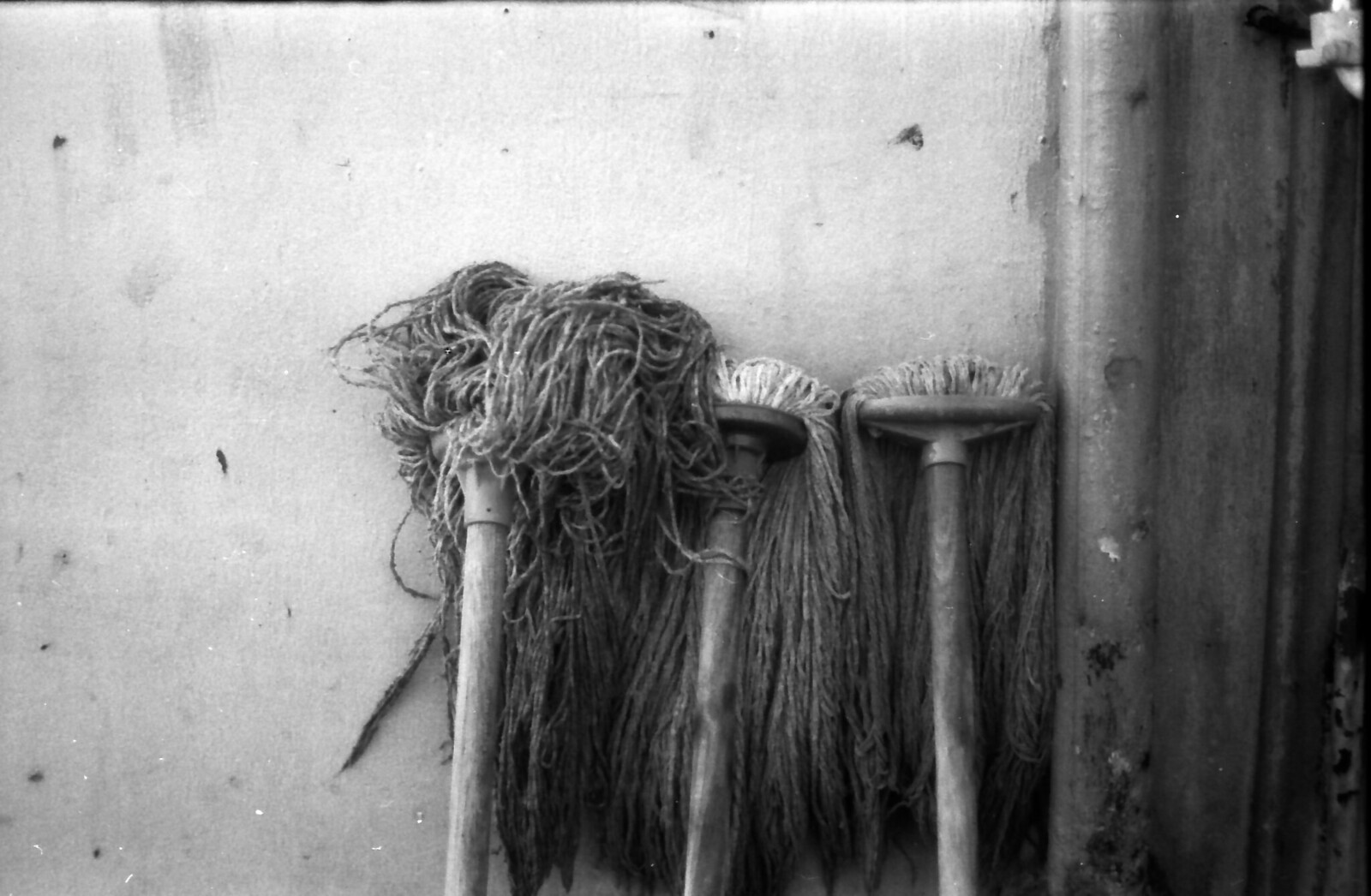This detailed black and white photograph, presented in landscape orientation, showcases an aged, worn wall made of stone or concrete, characterized by pockmarks and black stains, hinting at its long history. Leaning against this weathered surface are three mops, appearing significantly used. The mop on the left features a thick, "noodley" mop head resembling tangled spaghetti, mounted on a sturdy, wide cylindrical pole. The two mops to its right have narrower handles and cascade down the wall with their mop heads—one circular and the other rectangular. These mops appear newer compared to the first due to their smoother, more flowing strands. There’s a cylindrical beam fused to the wall, and to the far right, the concrete starts to break away into a shadowy area that's hard to discern. The background includes the faint outline of what might be a wooden panel or doorway, adding to the scene’s vintage character.